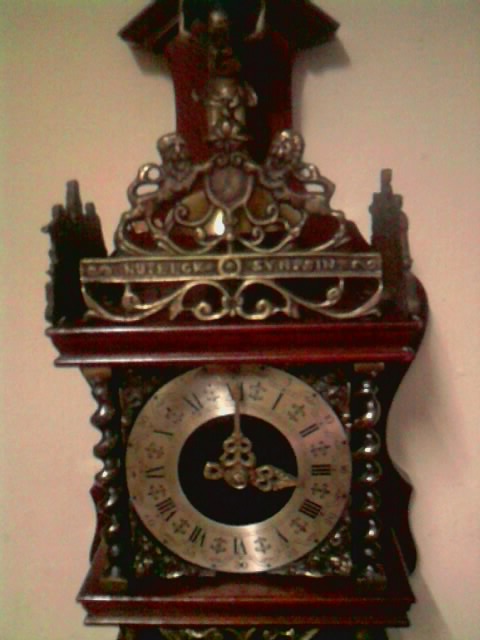The image is a detailed, close-up photograph, taken in portrait orientation, of an ornate clock, possibly a grandfather or pendulum type. The clock's elaborate design features a wooden body with intricate carvings, complemented by gold and other metal elements sculpted into the structure. The photograph captures a segment of the clock, with the top and bottom slightly cut off, leaving some ambiguity about whether it is freestanding or wall-mounted.

The clock face is prominently centered in the image. It consists of a black inner circle encircled by a brass or gold metal ring, resembling a doughnut. The ring is inscribed with Roman numerals in black, with the 12 at the top, the 3 on the right, the 6 at the bottom (upside down), and the 9 on the left, accurately marking the hours. The time displayed is approximately 3 o'clock, indicated by two ornate hands—an hour and a minute hand. These hands are intricately designed, reminiscent of Victorian-era keys, each featuring elaborate loops and shapes, with the minute hand bearing a resemblance to cutouts of a butterfly or leaves.

The background around the clock face is dark green with intricate patterns of gray, brown, and dark red, adding depth to the overall image. Near the bottom of the clock, a dark green section is discernible, intersected by a horizontal red line. The clock's upper section is adorned with sculpted elements, possibly resembling lions or mythical creatures, with their "paws" touching in the center, beneath a red crest with horn-like protrusions. This highly detailed, artistic timepiece exudes an air of historical grandeur and craftsmanship.